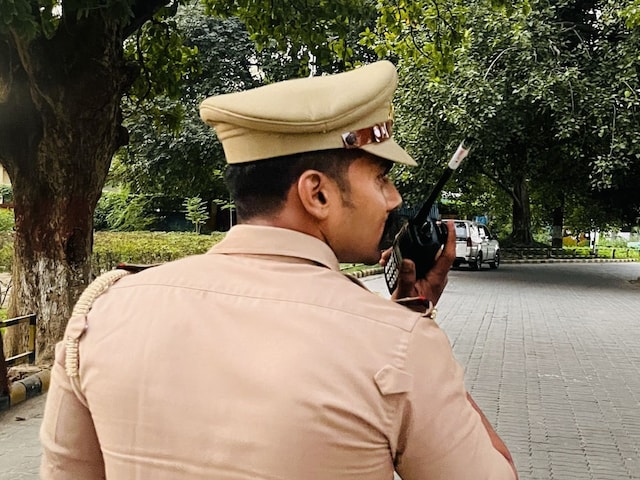The color photograph captures a man who appears to be a police officer or military personnel, wearing a distinctive tan uniform. His attire includes a tan half-beret, half-cap, and a fold-up collar on his beige, non-stretch cotton jacket, which has sleeves reaching to his elbows. Over his left shoulder, he wears a tan braided rope, suggesting a formal uniform. The man, sporting short black hair and sideburns, holds a black walkie-talkie in his right hand. He is positioned with his back to the camera, facing a pathway paved with gray bricks. Surrounding him is a lush green environment, with numerous trees including a notable large tree on the left side of the frame. A white truck is also visible in the distance, parked along the edge of the brick road.